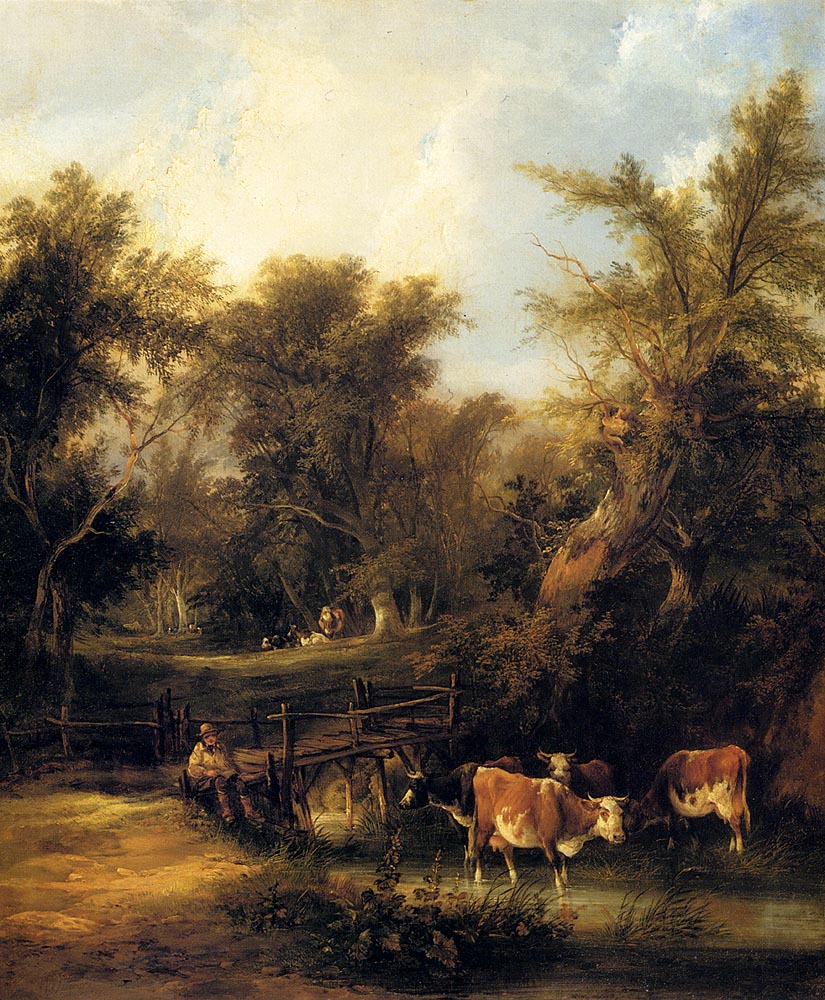The painting depicts a serene outdoor pastoral scene featuring a man seated on a wooden bridge, his legs dangling over the side, dressed in a wide-brimmed hat, light-colored jacket, and dark pants. Below him, four cows stand ankle-deep in a stream to his right: a black and white one with horns facing left, a brown and white one with horns facing forward, a white, brown, and white one with horns facing right, and another similarly colored cow facing left. Behind the man, a wooded area with dense, shadow-casting foliage extends across the scene. In a clearing within the woods, three more cows are visible—two lying down and one standing. The sky above is a vibrant blue, dotted with cloud matter, enhancing the tranquil atmosphere. The trees are described as bare in the middle but leafy at the top, creating dark, shaded patches under their canopy and over the field, suggesting a relaxing, somewhat sunny day.